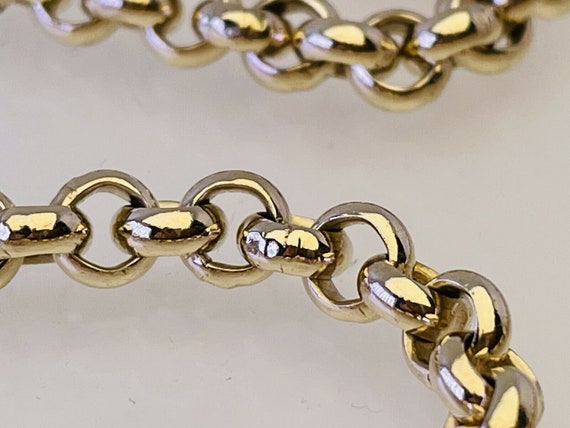In this highly detailed photograph, a close-up of a gold-linked necklace dominates the composition against a beige-off-white background. The image features two rows of interlocking circular links, with the primary focus on the lower chain that curves from the left middle of the frame to the bottom right. This prominent chain is perfectly crisp and shiny, highlighting its intricate craftsmanship. Above it, a second, slightly blurred row mirrors the first, extending from the upper left to the upper right of the photo. The interlocking circles in both chains alternate direction, creating a mesmerizing pattern. The reflection and shine of the gold links are evident, accentuating their luxurious appeal. No other objects compete for attention in this minimalist yet striking image.